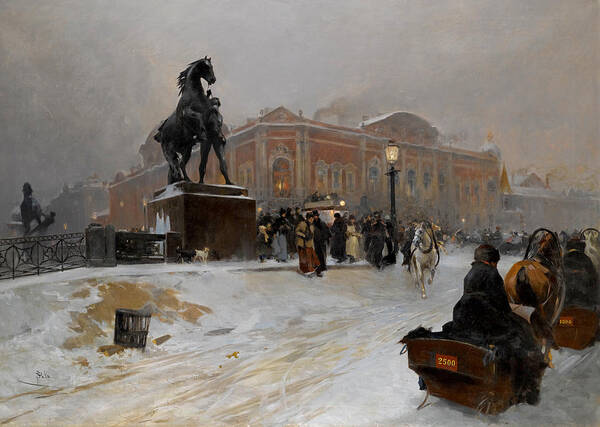The painting depicts a vibrant, snowy street scene set in St. Petersburg, Russia. In the foreground, the bottom right corner features several brown sleds, each pulled by horses. One sled prominently displays a gold placard with the number 2500 and carries a female rider draped in a black cape. Nearby, another similar sled pulled by a horse stands out.

Dominating the left side of the image, just above the middle, is a black statue of a rearing horse with a man holding its reins, positioned on a raised podium in a town square. A white dog stands alertly in front of this statue. The surrounding crowd, dressed in period costumes with long gowns and top hats, gazes up at the monument.

A white horse strides towards the viewer along the snow-blanketed street that angles from the bottom left to the top right. In the background, a grand, two-story reddish-brick building with cathedral-like arched windows and doors looms, adding to the sense of grandeur. The sky above is a mix of dark and light gray clouds, suggesting an overcast day yet with sufficient light to enhance the scene's clarity and vivid colors.